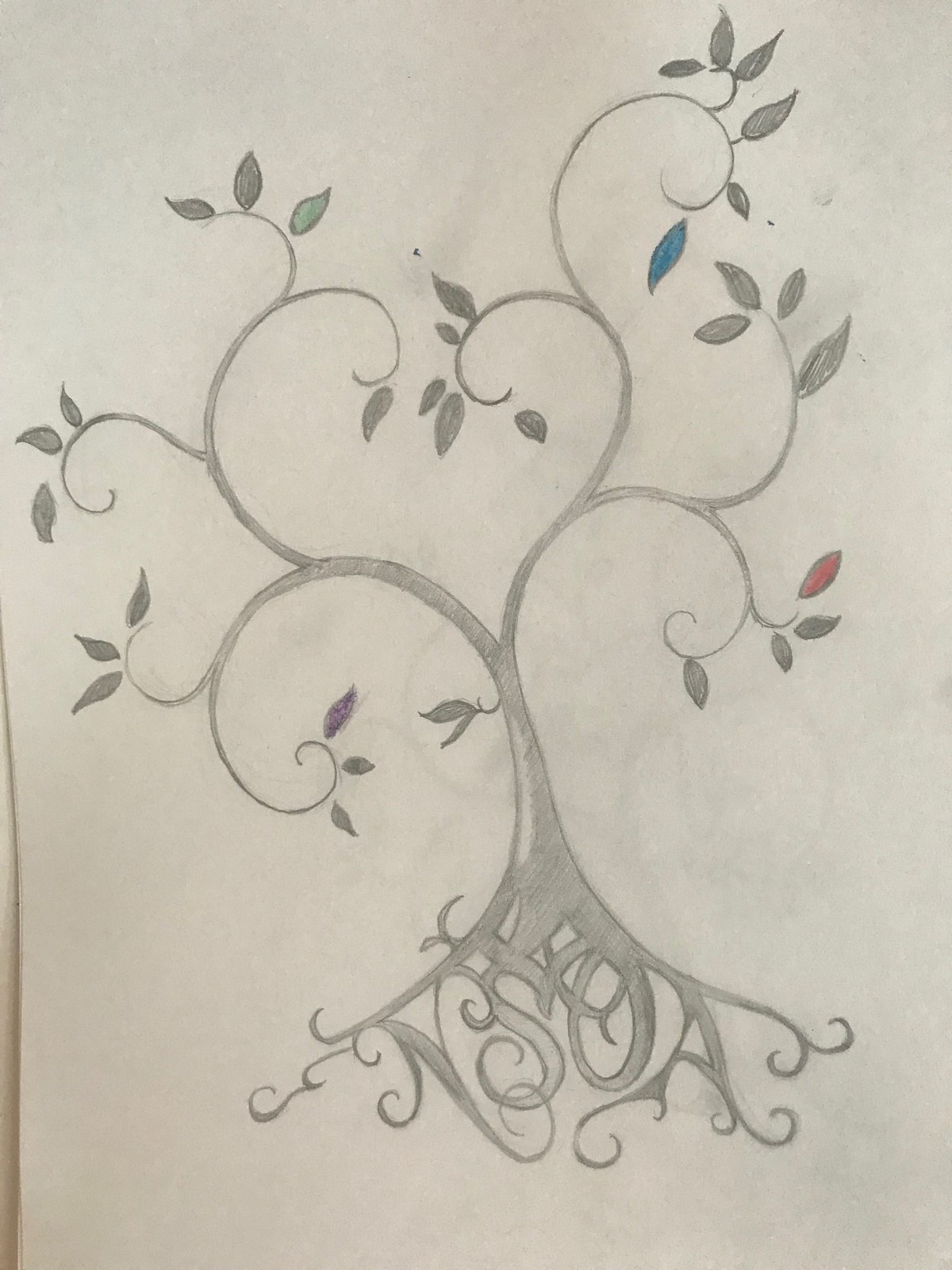This beautifully detailed pencil sketch depicts a thin-trunked tree with intricately criss-crossed roots that form the letters "N-S-O-A" in calligraphy-like style. The branches extend gracefully from the trunk, some curling into delicate curly cues that almost form the shape of a heart at the center. There is a harmonious blend of pencil-sketched leaves and sporadic touches of color, with some leaves shaded in blue or red. Each branch ends with a few sparse leaves, enhancing the tree's organic elegance. Set against a pristine white background, the artwork's intricate details and subtle touches of color make it a visually captivating piece, reminiscent of a family tree.